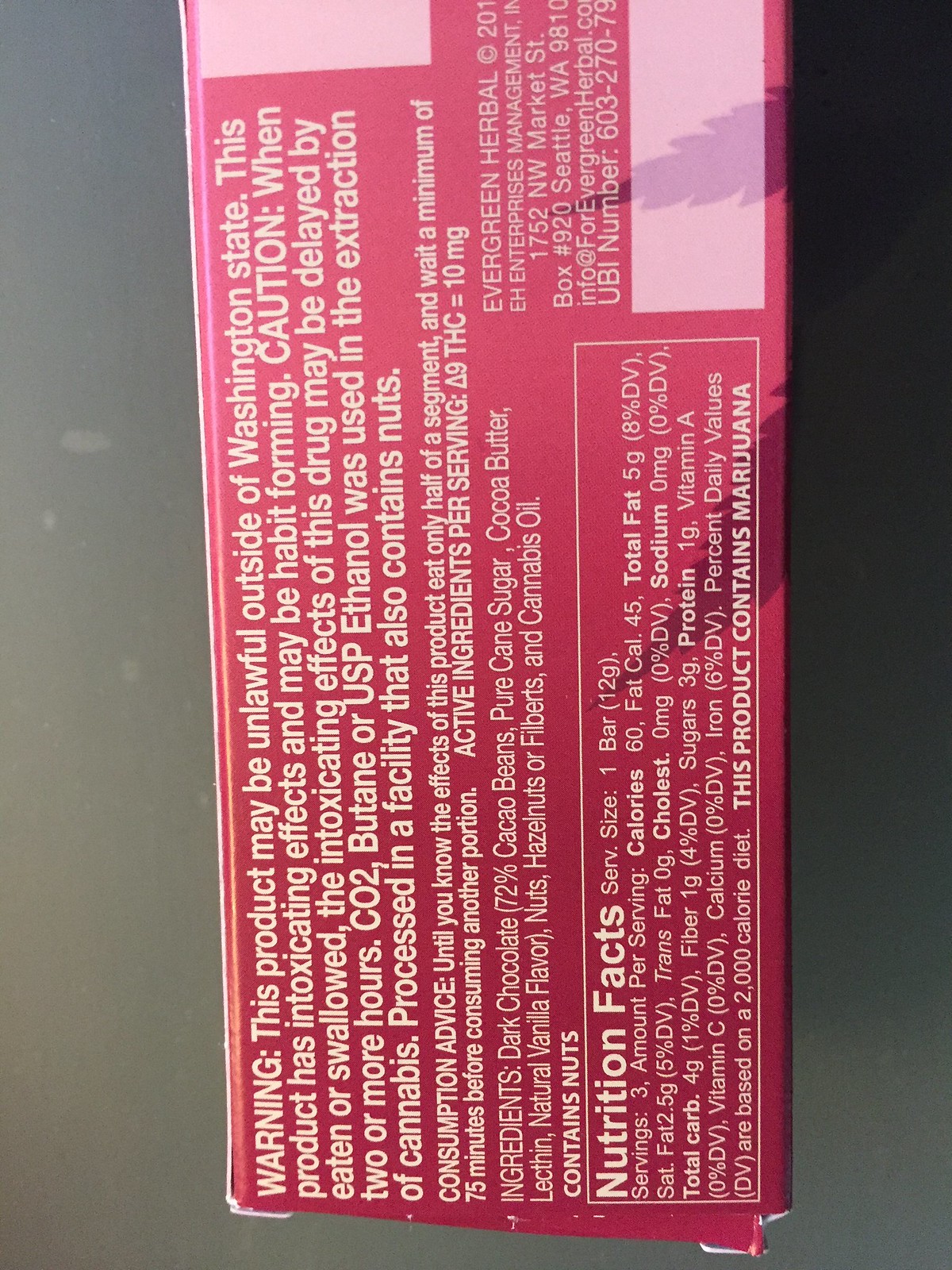The image showcases the back of a packaging for a THC-infused chocolate bar produced by Evergreen Herbal, based in Seattle, Washington. The packaging includes detailed nutrition facts and warning labels intended to inform the consumer about the product's ingredients and potential effects. The warning label prominently states: "Warning: This product may be unlawful outside of Washington State. This product has intoxicating effects and may be habit-forming. Caution: When eaten or swallowed, the intoxicating effects of this drug may be delayed by two or more hours." 

The extraction of cannabis for this product employed CO2, butane, or USP ethanol, and the facility also processes nuts. The nutritional information lists a serving size of 1 bar (12 grams), containing 3 grams of sugar, 1 gram of protein, and 0 milligrams of sodium. An essential advisory note urges consumers to "eat only half of a segment and wait a minimum of 75 minutes before consuming another portion" to gauge the effects.

The active ingredient per serving is delta-9 THC at a concentration of 10 milligrams. The bar's ingredients include dark chocolate, cane sugar, cocoa butter, and nuts. Clearly marked in bold letters, the package indicates that the product contains marijuana. The packaging is a red cardboard box, designed to safely contain the THC-infused chocolate bar while providing all necessary consumer information.